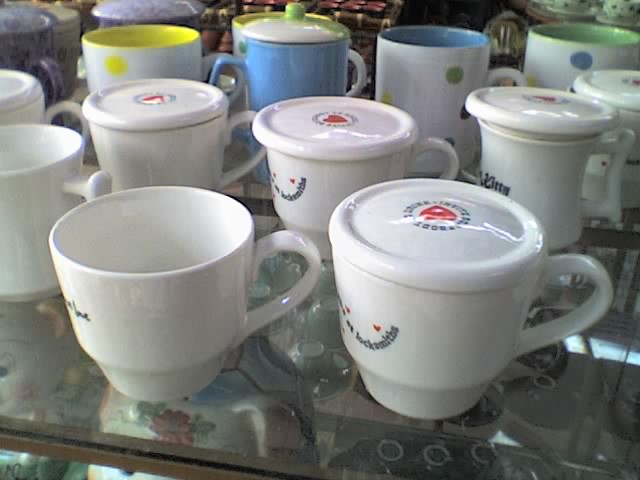This is a close-up photograph of a clear glass shelf with a dark brown wooden border, displaying an assortment of teacups and mugs. The white, glossy teacups are prominently featured, each adorned with small red hearts and indecipherable black text, some of which are positioned with their handles facing left, providing a side view. Among these are five similar-looking mugs with lids, each topped with a heart and bearing characters encircling it, while small hearts and text in a smile shape decorate the front. In the background, there is a variety of colorful mugs, including a white one with yellow polka dots, a blue one with a white top, and three white mugs with multicolored polka dots—each with a different interior color: yellow, blue, and green. The assortment of mugs, varying in shapes and sizes, evokes the organized display often seen in stores, reminiscent of Japanese shops like Daiso.